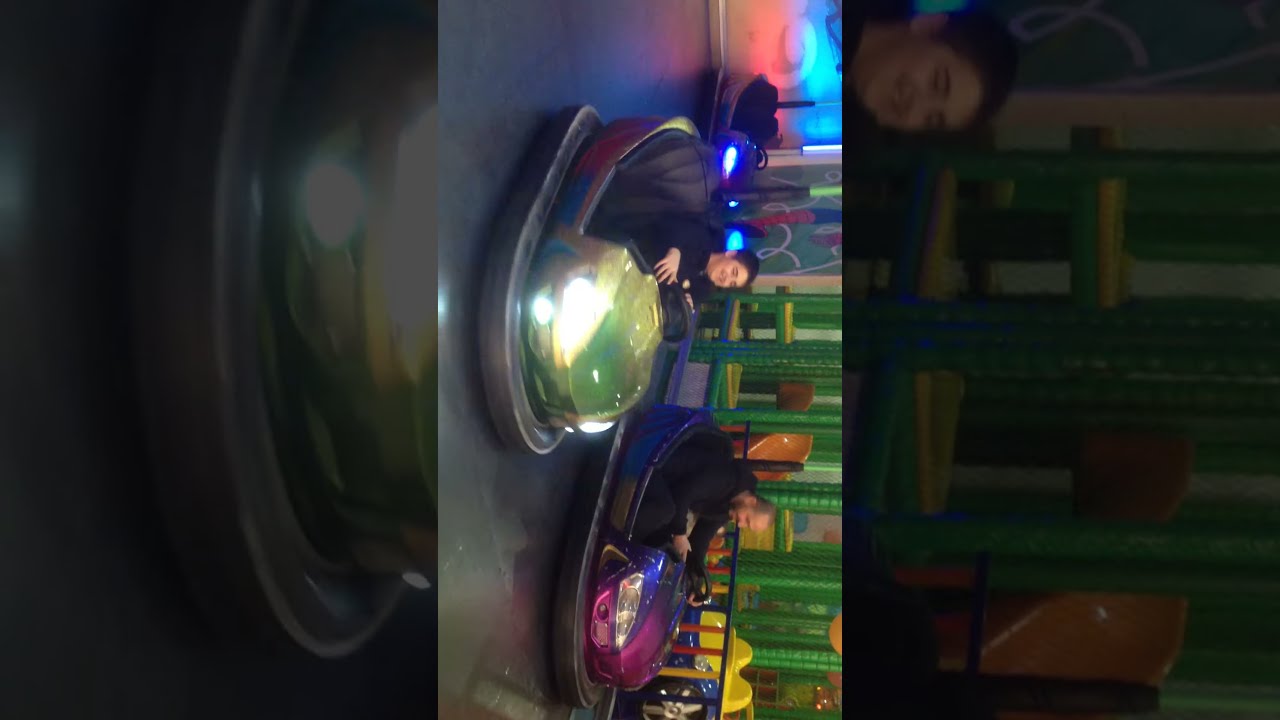In this vibrant and colorful image, originally taken vertically but displayed sideways, we see a lively indoor bumper car arena with a smooth, dark gray floor. At the center, there are two individuals joyfully riding bumper cars. On the left, a young boy with short black hair and a dark shirt is seated in a green bumper car with its headlights on, one hand on the steering wheel, and a smile on his face. To his right, an older man dressed entirely in black, with a very short shaved head and a mustache, grips the wheel of his blue and purple bumper car. The background features green walls adorned with colorful, illuminated decorations. Flanking the main scene, on the left, is a close-up of the front part of the green bumper car, slightly blurry and dark. On the right, there is a close-up of the boy's face with part of the green wall behind him. The image brims with a spectrum of colors, including blue, red, gray, green, yellow, purple, pink, and orange, enhancing the lively and fun atmosphere.